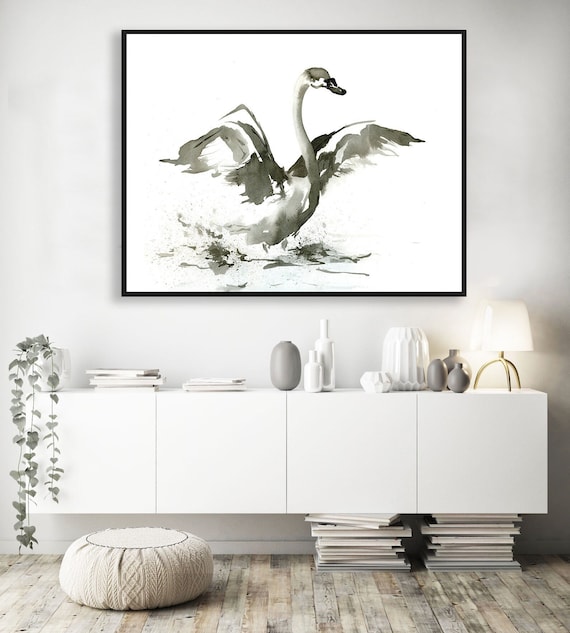The image depicts a modern, tastefully decorated room with a rectangular photograph that is taller than it is wide. At the bottom, there is a wood or faux wood floor, which extends underneath a sleek, white floating cabinet along the wall. The cabinet's design includes four square segments and rests on square ceramic slates, emphasizing a contemporary aesthetic.

To the right side of the image and beneath the cabinet, there are two stacks of magazines or records, creating an impression that they partially support the cabinet, though it floats independently on the left. Adding to the room's cozy ambiance, a small round seat pillow or ottoman is placed on the left side of the floor.

On top of the cabinet, there are several decorative items, including small vases and vessels in gray and similar muted tones. There is also a distinctive, short white lamp with a white lampshade supported by three curved legs, and a plant in a white pot. These items contribute to the sophisticated yet minimalist decor.

Dominating the wall space above the cabinet is an abstract black-and-white watercolor artwork of a swan, characterized by its outstretched wings. The overall color palette of the image is composed of soft hues of white, gray, and cream, lending the room a light, subdued, and serene atmosphere suitable for a magazine cover or interior design feature.